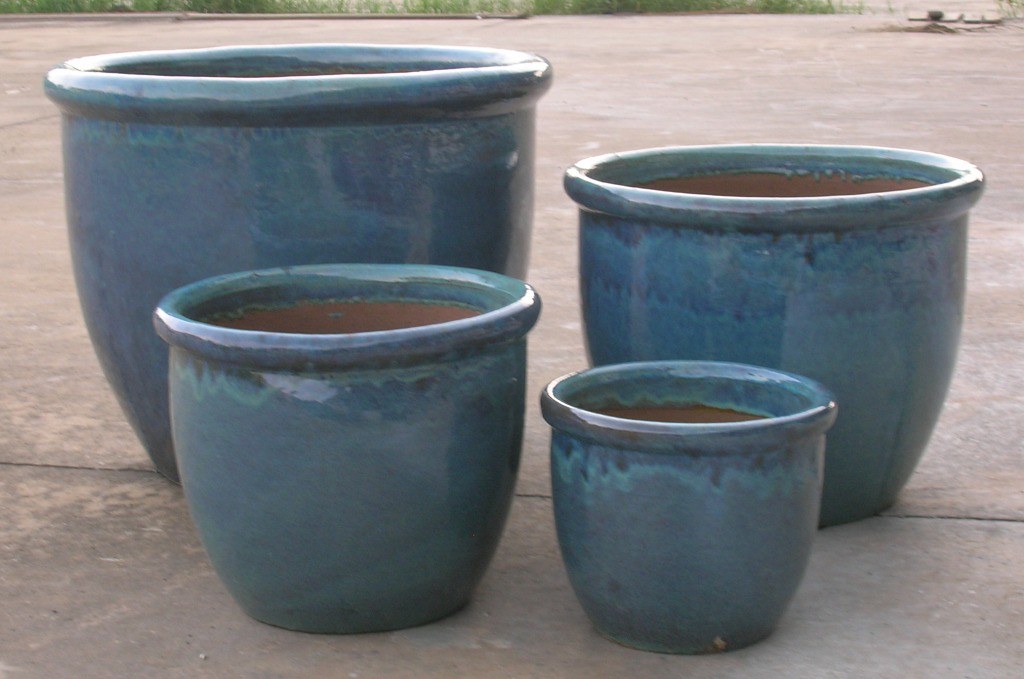This photograph features four terracotta pots, arranged on a reddish concrete patio in an outdoor setting. Each pot, coated in a shiny, multicolored blue glaze with visible drip marks and a textured finish, reveals a contrasting terracotta color on the inside. The largest pot sits in the back row on the left, followed by the second largest to its right. In the front row, the third largest pot is positioned on the left, while the smallest pot occupies the right front corner. The pots exhibit a slightly dusky sheen with hints of green and geometric effects resulting from the glazing process. A thin strip of green vegetation is visible at the very top of the image, suggesting a garden setting. The scene appears sunlit, highlighting the intricate details and vibrant hues of the pots. The pots, which appear to be empty, each feature a pronounced rounded lip at the top.